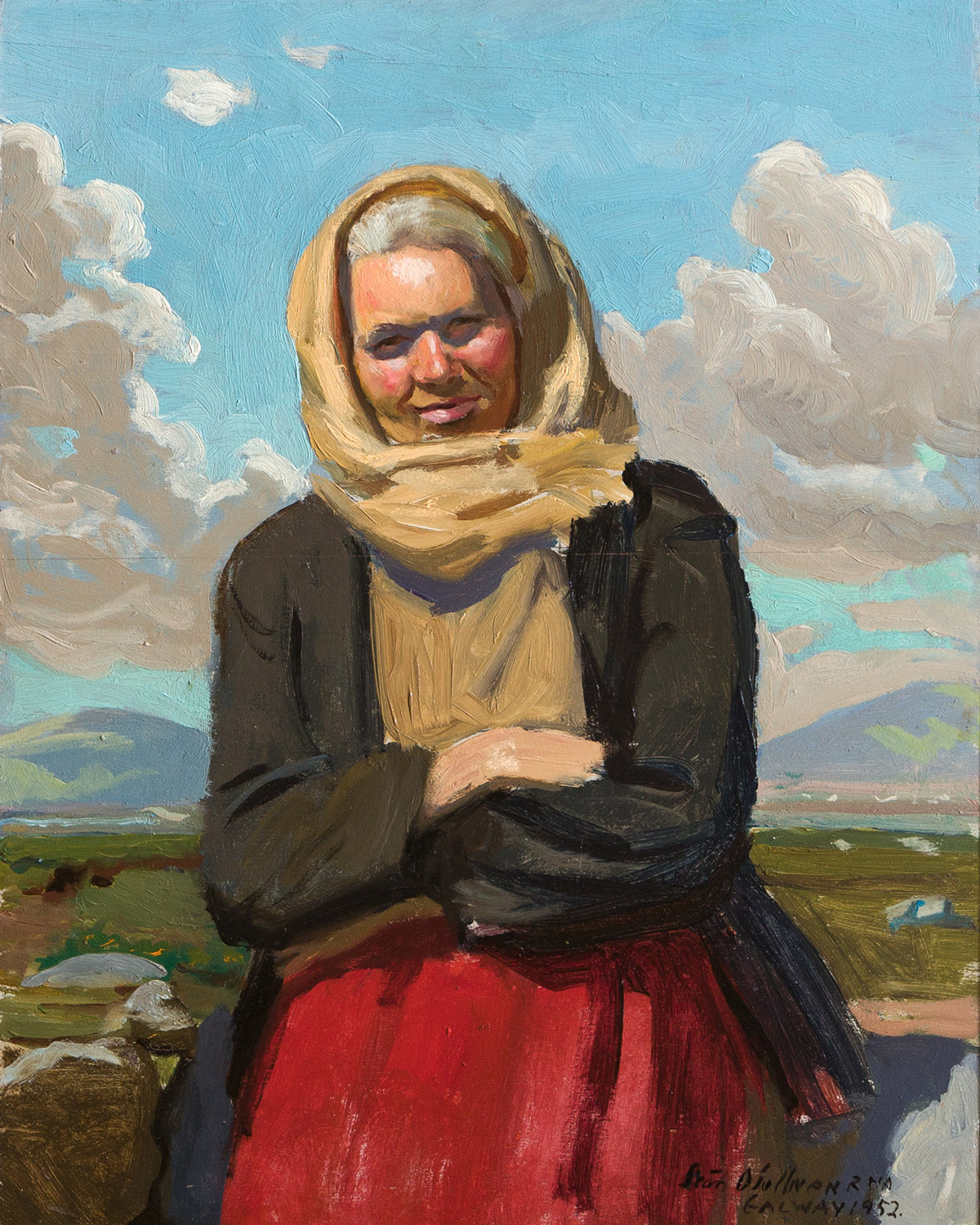This captivating piece of artwork by Dean Dewey, dated 1952 and rendered in a vertical orientation, combines acrylic and oil paint techniques. The painting features a Caucasian or European woman as its central subject. Her attire includes a beige scarf wrapped around her head in a style reminiscent of a hijab, revealing her gray hair. She wears a black long-sleeve cardigan over a beige sweater and a red long-sleeve dress. With her arms folded in front of her, she is depicted from above the knees, standing against a backdrop of a serene countryside.

Behind the woman stretches an olive-green field, leading up to a valley with majestic mountains. The sky above her is a brilliant blue, interspersed with stormy gray and white clouds. The subtle details, such as her tan skin, rosy red cheeks, and the bright quality of sunlight, enhance the vividness of the painting. Her expression, marked by a squint and a gentle smile, adds warmth to the scene. The artist's skillful brush strokes are visible, contributing to the painting's textured and lively appearance.